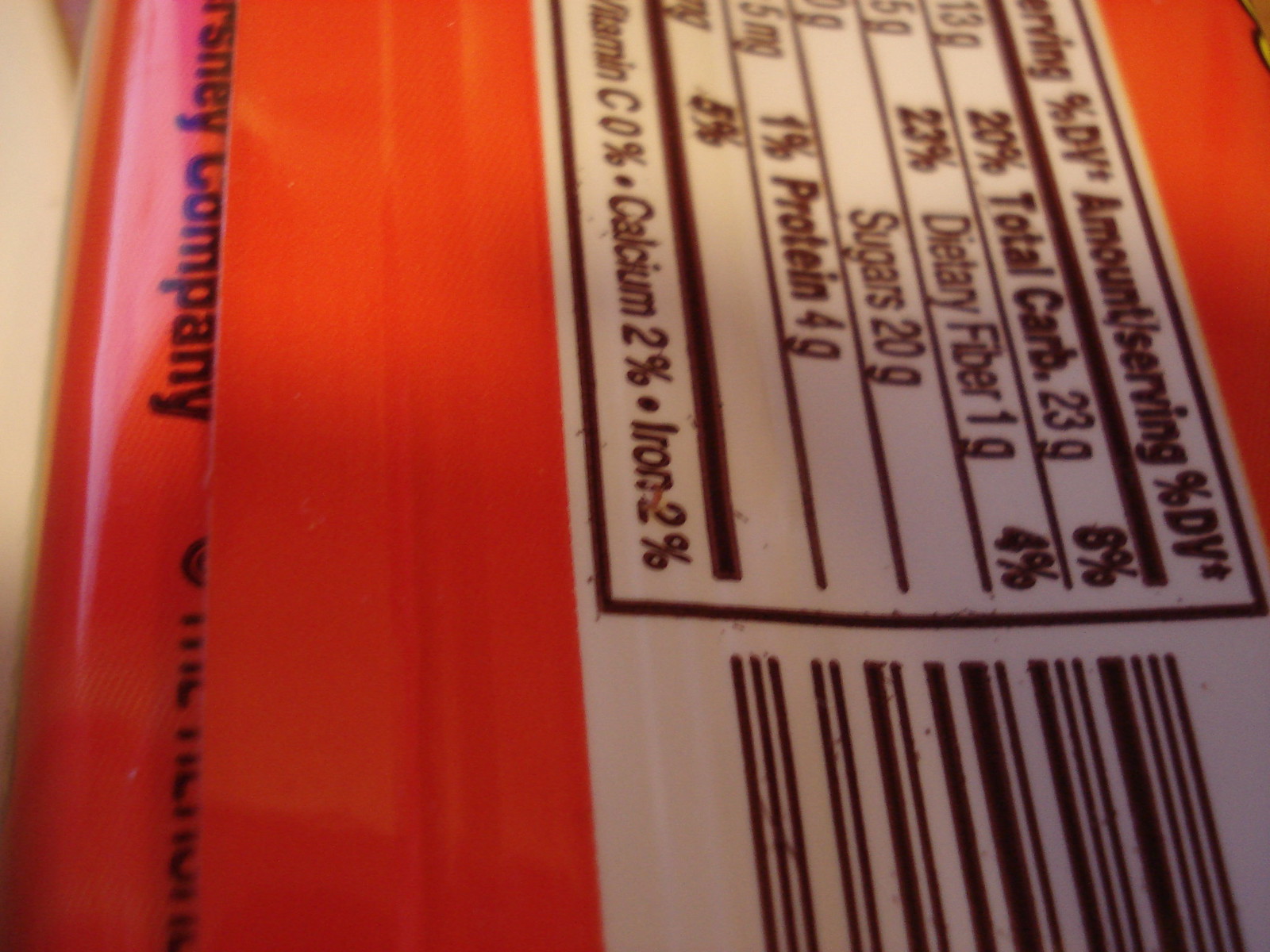This image is an up-close photograph of the nutritional label on what appears to be a Reese's candy bar, given the context and nutritional information. The packaging is a distinctive orange, with the label displayed vertically, meaning the words are sideways. The right side of the label indicates the barcode, while nutritional details such as total carbohydrates (23 grams or 8% daily value), dietary fiber (1 gram or 4% daily value), sugars (20 grams), and protein (4 grams) are clearly visible. The label's white background and dark lettering contrast sharply against the orange of the packaging. A small flap partially obscures text at the top left, revealing only "company" and part of "S-H-E-Y," suggesting it refers to the Hershey Company. Additionally, the label specifies that the product provides 2% of the daily values for both calcium and iron.